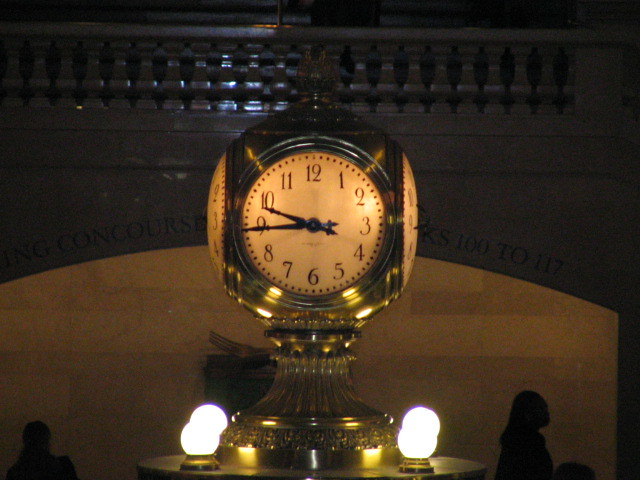The image depicts the interior of a New York train station, featuring an abundance of vertical posts arranged in rows along the concourse. The back wall is adorned with elegant stone tiling, giving a grand and timeless feel to the setting. The floor is dappled with shadows cast by silhouettes of people, primarily concentrated on the left and right sides of the frame.

Prominently in the center stands a stately clock mounted on a platform. This clock boasts an intricate design, where its base elegantly narrows into an hourglass shape before expanding into a spherical top. The clock face is bordered with dot markers around the numerals, and it displays the time with an hour hand nearing the 10 and a minute hand approaching the 9. The clock and its components exhibit a lustrous brass metal color, adding a touch of vintage charm. Surrounding the platform are large lantern-style lights with substantial bulbs, further illuminating the scene and enhancing the station's ambiance.